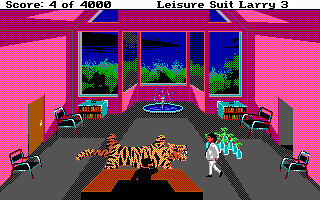An in-game screen with a score of 404,000 from the game "Leader Suite Larry 3." The room features vividly bright pink walls, adorned with windows offering a captivating view of water—possibly a river or ocean—flanked by trees. Dominating the room is a small fountain with visibly flowing water. In the middle of the scene stands a large, roaring Bengal tiger facing a person approaching it, while another individual stands behind a wooden desk. The room also contains four chairs, a wooden door, and appears to be part of a large office or spacious environment, complete with a bookshelf in the background.